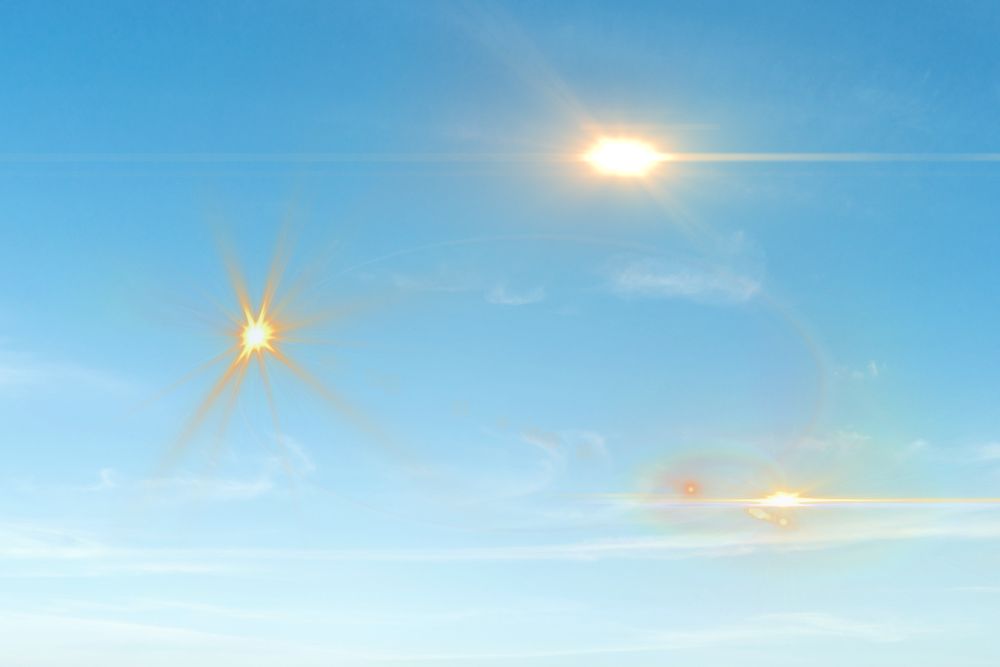The image captures a vast, light blue sky that fades to a cloud-like whiteness towards the middle and bottom. Within this ethereal scene, there are multiple bright, sun-like bursts of light. The most prominent burst occupies the upper left portion of the image, emanating a radiant combination of yellow, white, and orange hues, resembling a starburst. Below this, toward the right middle portion, a smaller, elongated sun-like burst stretches horizontally in a flattened manner, extending far left and right. A third, smaller but impactful burst can be seen in the lower right, emitting rays of yellow light horizontally across the sky. Altogether, the image conveys a surreal and celestial atmosphere, with these luminous projections creating an intriguing and almost cosmic tableau.